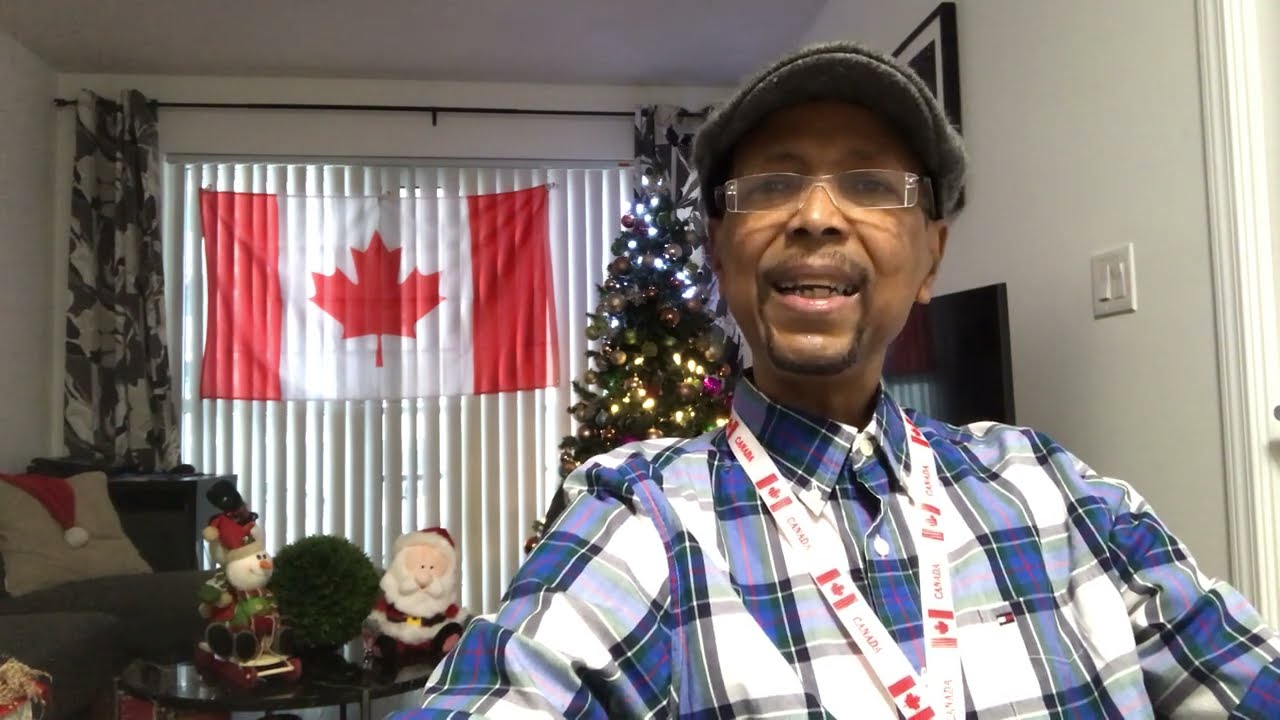In the image, an older African-American gentleman is seen wearing clear glasses, a gray woolen cap, and a lanyard emblazoned with the Canadian flag and the word "Canada." His attire includes a plaid shirt with white and blue patterns accented by subtle red stripes. The man, who sports a goatee, is seated and facing the camera. Behind him, the festive spirit is evident with a brightly lit Christmas tree situated near his head and right shoulder. Additional holiday decor includes stuffed Santa Claus and snowman figures on a coffee table, and a Santa hat draped over the back of a gray couch. A Canadian flag adorns a sliding glass window with drawn shades in the background. The surroundings of the house, marked by white walls and ceiling, also feature a turned-off flat-screen TV positioned near the man's right ear. The setting unmistakably suggests a cozy Canadian Christmas scene.